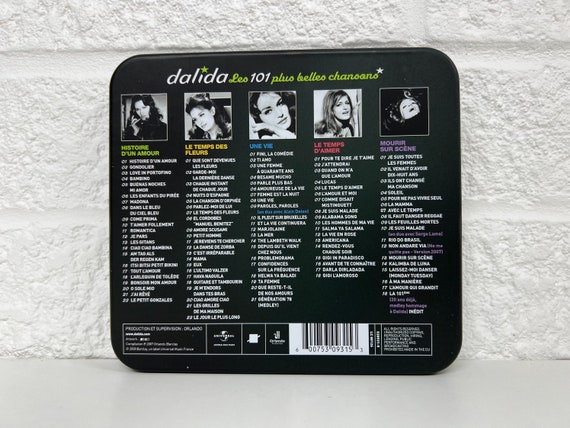This image depicts the back cover of a CD, primarily in Spanish. At the top, the title "Delita" is prominently displayed in white letters, with a green star substituting the dot over the 'I'. Below "Delita", the name "Leo" is written in green cursive lettering, followed by "101" in white lettering, and then "Pueblo Chonona" in green cursive writing. The central portion of the cover showcases five square pictures of women, likely representing different artists. Beneath these images, there are columns of white-lettered text enumerating song titles and names, possibly album titles. The listed titles include "Historie d'un amour," "Les temps d'effluves," "Une vie," "Les temps d'années," "Mont-Cézanne," among others. Towards the bottom right, slightly off-center, there is a UPC barcode accompanied by additional informational text. The entire layout combines details and structuring to highlight the variety of content included on the CD.